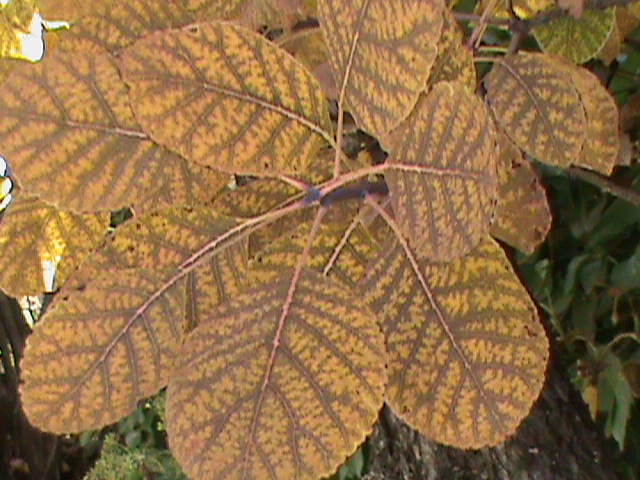This detailed photograph captures a close-up view of a tree branch adorned with vivid autumn leaves in various stages of transformation. Dominantly, the leaves exhibit a range of golden-yellow to brown hues, interspersed with touches of pink, beige, and hints of green from the background foliage. The leaves, teardrop to oval in shape, display intricate vein patterns and some have small holes, likely the work of hungry insects, adding texture to the scene. The photograph's composition is dense with layers of leaves, allowing for the sunlight to dapple through, casting a gentle glow that enhances the autumnal palette. Behind the primary cluster of leaves, one can discern the green leaves and brown bark of the tree, providing a contrasting backdrop. Branches and stems, some in shades of pink and dark brown, crisscross the image, adding depth and framing the leaves. The overall atmosphere evokes the crisp transition of fall, with bright lights from behind emphasizing the season's rich, warm tones.